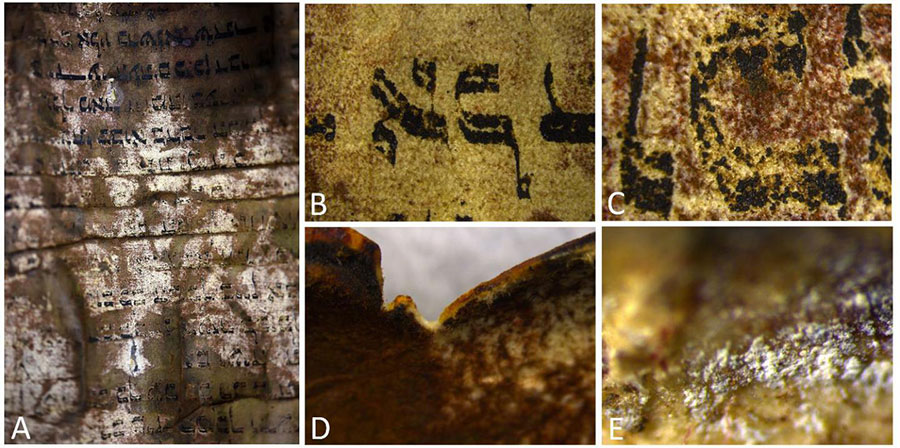This collage image features five individual pictures labeled A through E, each depicting ancient manuscripts and their text. Image A presents a distant view of ancient Hebrew text on a severely weathered, brown and white parchment, showcasing its distressed condition. Image B offers a closer examination of the Hebrew characters, revealing intricate brush strokes on the similarly battered surface. Image C zooms in even further, emphasizing the detailed wear on the parchment and the intricacies of the characters. Image D deviates slightly, displaying a visually striking textured area resembling a red and burgundy ridgeline, perhaps part of the manuscript or an associated artifact. Lastly, Image E provides an extreme close-up view, capturing a texture that appears almost microscopic, with visible fragments and a mix of brown, black, and gleaming particles, likely highlighting the physical composition of the ancient writing surface.